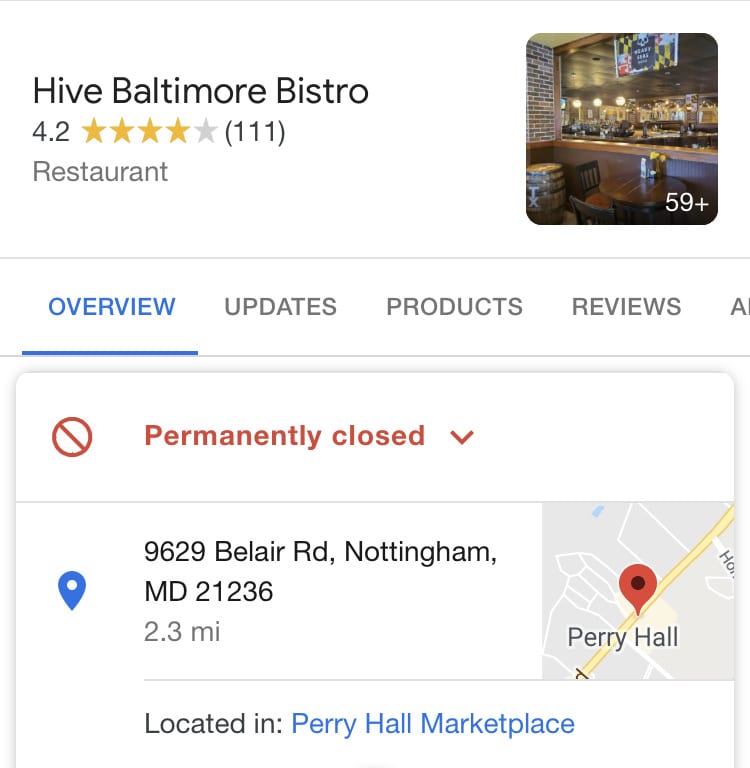Screenshot of a Google Maps search for Hive Baltimore Bistro, a now permanently closed restaurant. At the top of the page, the restaurant is listed with a rating of 4.2 stars based on 111 reviews. The restaurant was located at 9629 Bellaire Road, Nottingham, Maryland, 21236, within Perry Hall Marketplace. The "Overview" tab is selected and highlighted in blue, indicating the status of the establishment as "permanently closed." The page also mentions additional details and reviews under various tabs such as "Updates" and "Product Reviews," but they are not selected. A photo of the bistro is visible, with an indication that there are 59 more images available. Regrettably, as per the information from Google, this dining spot has ceased operations, leaving its patrons to seek alternative venues.